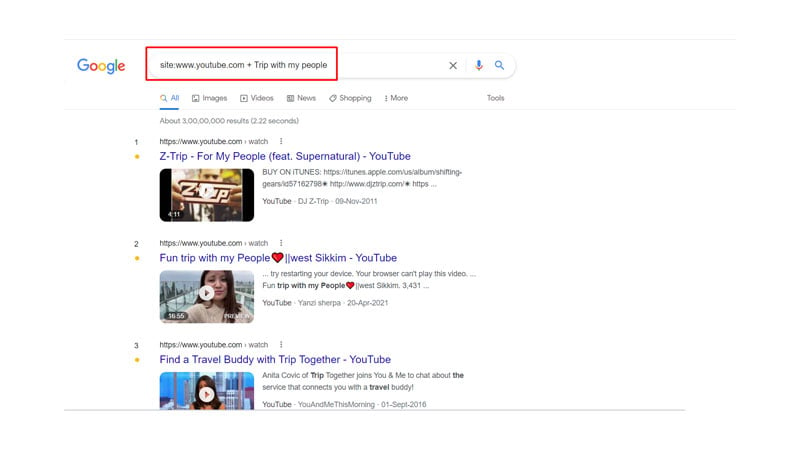A Google search has been conducted with the keywords "site:www.youtube.com trip with my people." The search box containing these words is conspicuously highlighted in red. Below the search bar, all the text is selected, indicating that it is ready for editing or modifying. The search query has yielded over three million results. 

Displayed on the screen are three specific search results:
1. The first result is a video titled "Z-Trip for my people featuring Supernatural."
2. The second result is an article or video titled "Fun trip with my people, West Sikkim."
3. The third result appears to be a video with a partially visible thumbnail, depicting about two-thirds of the image, and is titled "Find a travel buddy with Trip Together."

Each result potentially relates to different content types, including music, travel experiences, and social travel platforms.